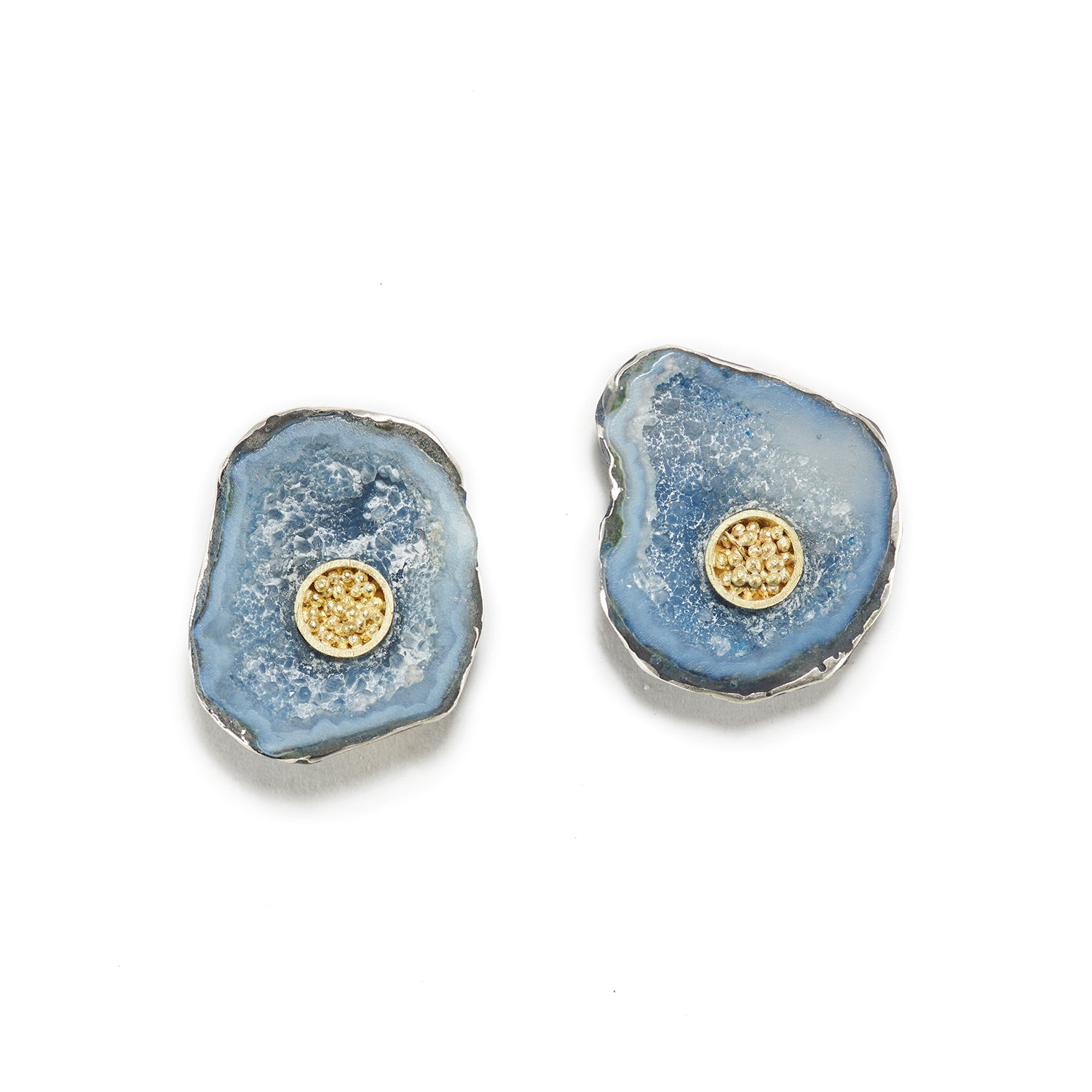This image portrays two geological rock halves, suggestive of the inside of a clamshell, positioned side by side. Each half resembles part of an oyster, with a striking outer layer of dark charcoal gray blending into hues of bluish gray. The interior is a mesmerizing light blue, interspersed with sparkling white and blue crystal formations, giving the rocks a gem-like appearance. Both halves feature a prominent, centrally located, golden ring containing a cluster of small, shimmering golden beads, which create a stark and intriguing contrast against the crystalline background. This composition captures a unique blend of natural rock formations with artistic embellishment, emphasizing the beauty of both the earth’s geological wonders and human creativity.